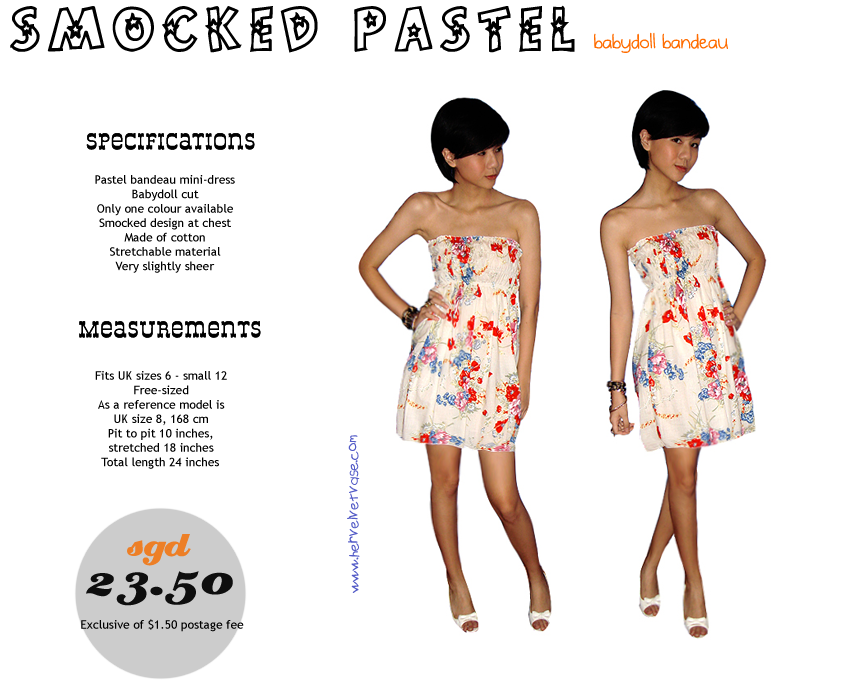The advertisement features an Asian girl with short black hair modeling a smocked pastel babydoll bandeau dress. The dress is strapless, predominantly white, and adorned with a pattern of red, blue, and pink flowers. The model is depicted in two different poses: in one, she stands with her right hand on her hip and her legs crossed, looking over her shoulder; in the other, she has her left hand on her hip, and her right arm hangs by her side as she looks into the camera. At the top of the image, the text reads "Smocked Pastel Babydoll Bandeau" in black and orange letters. On the left side of the image, detailed specifications describe the dress as a pastel bandeau mini dress with a babydoll cut, available in only one color, featuring a smocked design at the chest, made from stretchable cotton material that is very slightly sheer. The measurements indicate it fits UK sizes 6 to small 12, with the reference model being a UK size 8, 168 centimeters tall. The dress has a pit-to-pit measurement of 10 inches that stretches to 18 inches, and a total length of 24 inches. The price is listed as SGD 25.30, exclusive of a $1.50 postage fee.